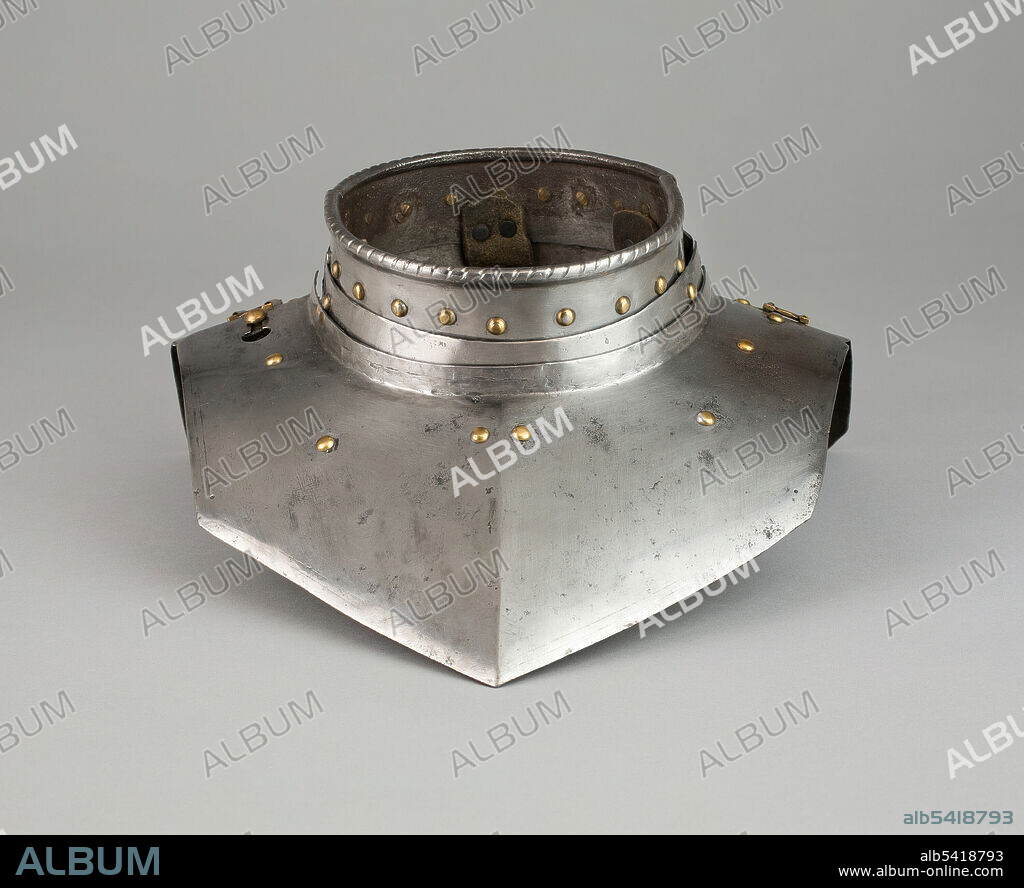This image showcases a detailed side view of a medieval neck piece crafted from steel, adorned with gold-toned rivets spaced about an inch apart around the collar. The neck piece extends over the clavicle to the tops of the shoulders and is pointed at the front. Notably, it features two metal rings below the neck, suggesting that a mouthpiece could once have been attached. The steel is aged, displaying patches of black tarnish, indicating its antiquity. The background of the image is gray, and across it is a repeated watermark that reads "ALBUM" in gray and light gray. At the bottom of the photo, a thick black rectangle spans the width, with "ALBUM" in blue on the left. On the right side of the rectangle, the identification number "ALB5418793" and the URL "www.albumonline.com" are displayed in white text. These details comprehensively capture the intricate features and historical significance of the neck piece, framed within the labeled and watermarked context of the photograph.